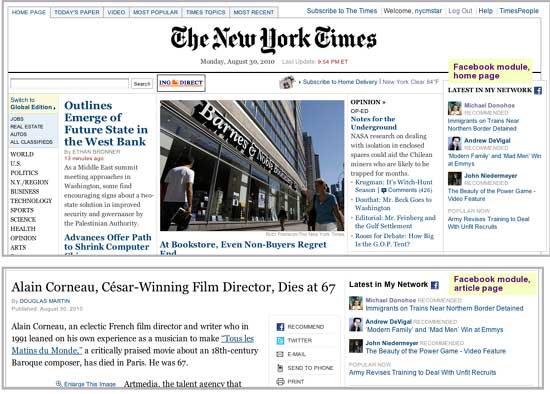A detailed screenshot of the New York Times website reveals its classic interface. At the top, several navigational tabs are displayed in a small, delicate font, challenging to read but identifiable as links to the Home Page, Today's Paper, Video, Most Popular, Times Topics, and Most Recent sections. Appearing as white tabs with blue font, these options provide quick access to different areas of the site.

To the right of this menu, additional options include Subscribe, Popular, Logout, Help, and Times People, offering a range of user interactions. Centralized on the page, the iconic "New York Times" logo is prominently displayed in its traditional newspaper font. Below the logo, the current date is printed, followed by a sharp, black horizontal line that delineates the navigational features from the content area.

In the content section under this line, a central photograph of a Barnes & Noble storefront captures attention. To the left of the photograph, a headline reads "Outlines Emerge of a Future State in the West Bank," though this article is unrelated to the bookstore image. Directly beneath the photograph, an article titled "At Bookstore, Even Non-Buyers Regret" delves into the narrative associated with the image.

To the right of the content, a sidebar features a section titled "Latest in New York Networks," providing updates and links to new stories. Below the main article, an obituary headline announces "Alain Corneau, César-Winning Film Director, Dies at 67," adding a somber note to the news snapshot.

This comprehensive screenshot encapsulates the blend of news, opinion, and cultural touchpoints that visitors to the New York Times website can expect.